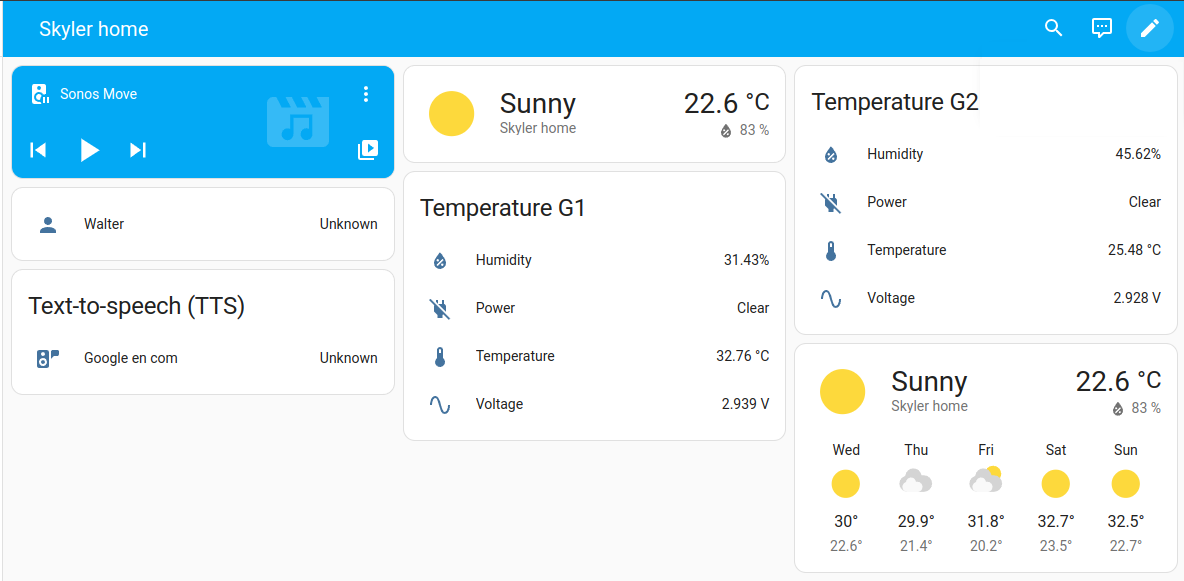Here is a cleaned-up and detailed caption for the image described:

---

The image is a screenshot featuring several informational banners and icons against a bright sky blue background. 

At the top left, the text "Skyler Home" (capitalized as S-K-Y-L-E-R H-O-M-E) is prominently displayed. Moving to the right, there are three white icons: a magnifying glass, a chat bubble with three dots inside, and a light blue circle containing a pencil. 

Below these, a banner on the left side reads "Sonos Move" (capitalized as S-O-N-O-S M-O-V-E), accompanied by icons for rewind, play, and fast forward. A music note icon appears underneath.

Further down, another banner displays the text "Walter" with the word "Unknown" on the right. Beneath this, yet another banner states "Text-to-Speech (T-T-S)" with the text "Google EN Com" and "Unknown" on the right.

Adjacent to these on the left, a detailed weather and environmental information panel is shown. It reads:
"Sunny in Skyler Home, 22.6 degrees Celsius, 83% chance of precipitation." Below this, specific metrics are provided:
- Temperature G-1: 31.4 (30% Humidity), Power status is clear, Temperature 32.76 degrees Celsius, Voltage 2.939 V.
- Temperature G-2: 45.62% Humidity, Power status is clear, Temperature 25.48 degrees Celsius, Voltage 2.928 V.

At the bottom, the days of the week—Wednesday through Sunday—are listed, indicating ongoing sunny weather at Skyler Home.

---

This caption provides a comprehensive and structured description of the screenshot.